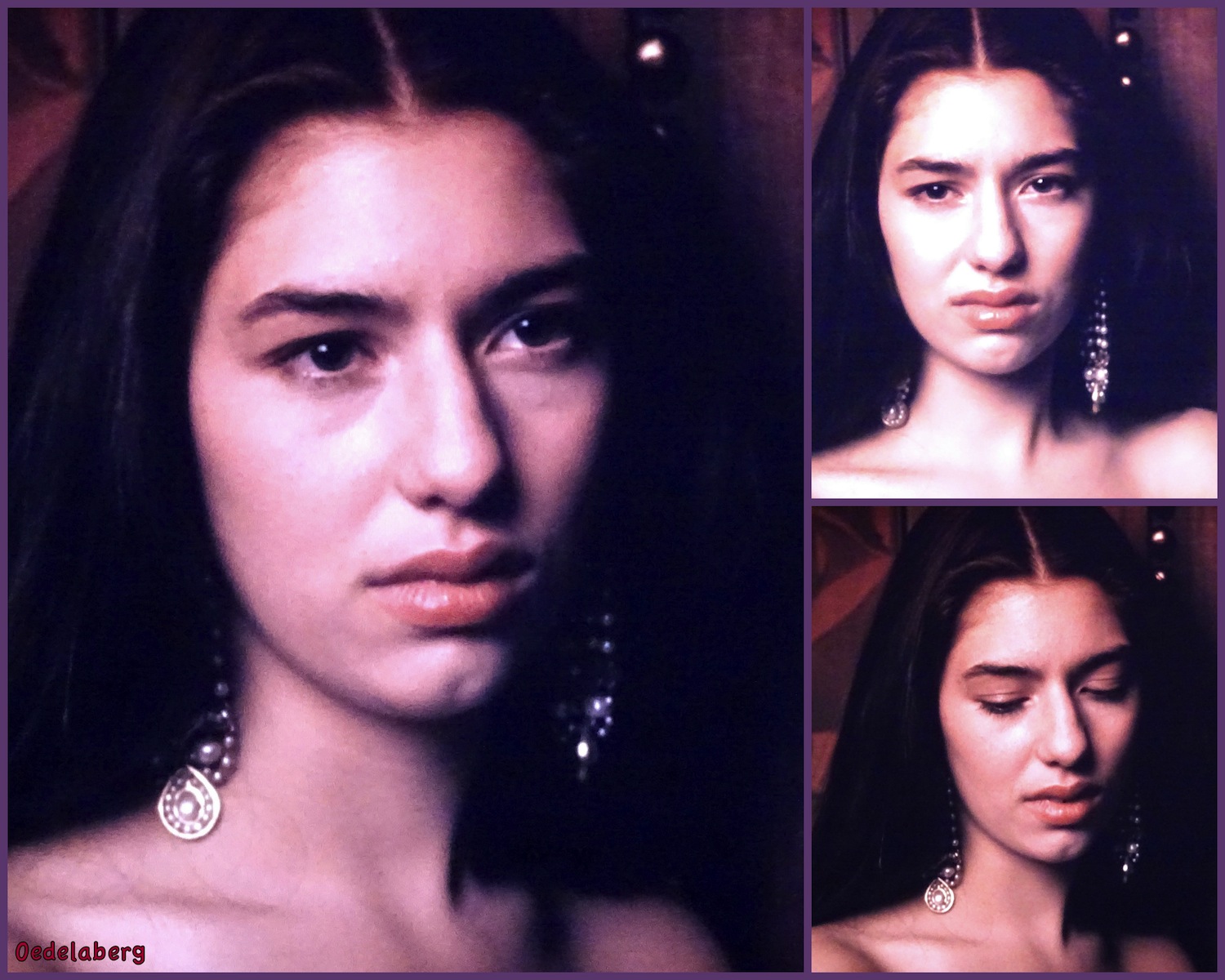The image is a composite featuring three shots of a young woman who might be Coppola's daughter from The Godfather. In a three-tiered layout, the primary image occupies the left two-thirds of the frame, showing the woman with tanned skin and long, middle-parted black hair. She wears long, dangling earrings with pearl-like stones, and her expression suggests sadness or irritation. Her lips are pursed, and her torso is mostly nude, except for a partially visible dress. 

The top-right photo, smaller than the main one, captures the same woman staring directly at the camera with a decidedly unimpressed look on her face. The bottom-right image shows her with her head tilted downward, eyes almost closed, and still wearing the same earrings, though partially concealed by her hair. All three photos share a dark background and convey a consistent mood of discontent or unhappiness. Notably, red text reading "O-E-D-E-L-A-B-E-R-G" appears in the bottom left corner of the composite.